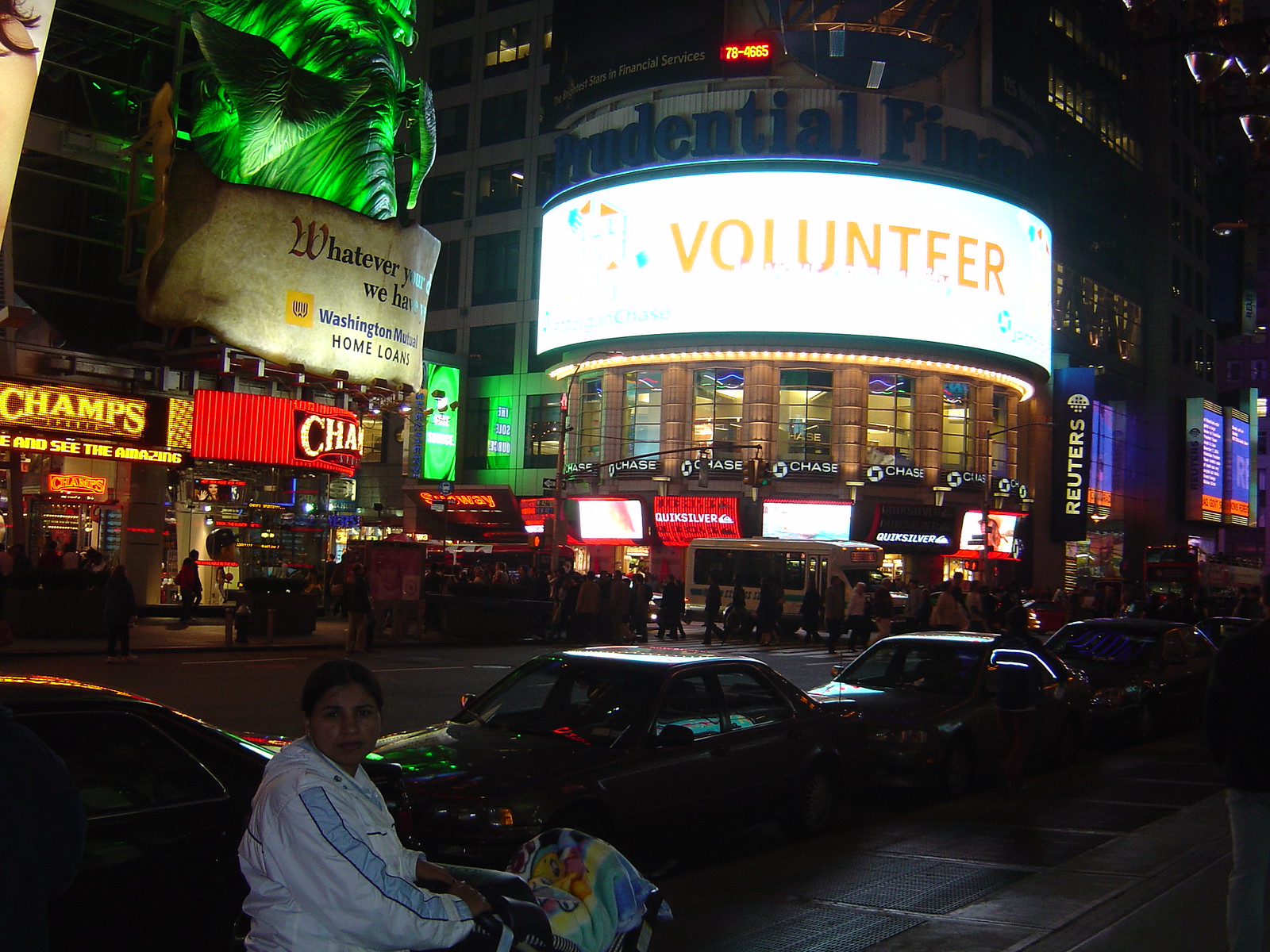The image depicts a vibrant, bustling city center at night, with a main focus on a prominent Prudential Financial building featuring a distinct round, rotunda-like facade. At the top of this building, a large, illuminated round neon sign displays the word "Volunteer" in gold letters on a white background, beneath which a non-illuminated "Prudential Finance" sign is visible. The building's windows are adorned with repeated Chase logos, advertising "the brightest stars in financial services" with the number 78-4665. The street is lively, with both parked cars and moving traffic, as well as pedestrians. Multiple other buildings and billboards surround the scene, including advertisements for Champs, Quicksilver, Reuters, and Washington Mutual Home Loans. A young man, possibly pushing a stroller, is in the foreground of the image. Despite the numerous neon signs, the street maintains a darker ambiance, primarily lit by the glowing advertisements above, suggesting a busy yet slightly mysterious urban environment, potentially reminiscent of New York City.